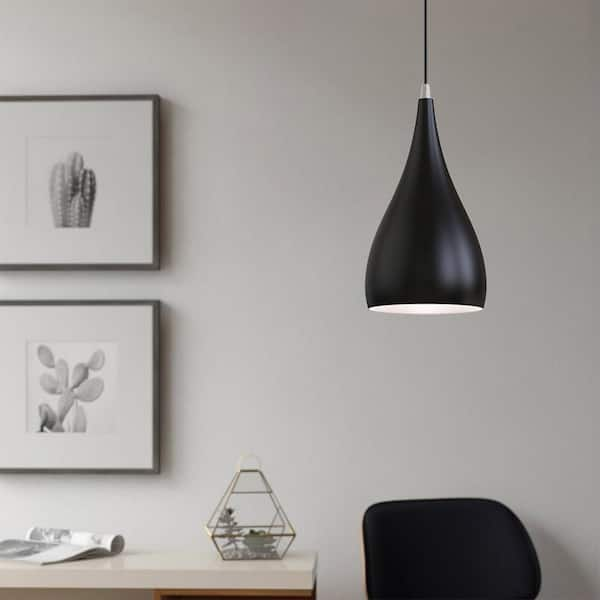The indoor image appears to be taken in a home office. The backdrop features solid white walls adorned with two square picture frames, each containing black and white photographs of cacti, bordered by dark gray frames with a white mat. Below these frames is a cream-colored desk, upon which lies an open black and white magazine. A desk ornament, possibly a small cage with a tree and bush, also decorates the surface. Suspended from the ceiling is a glossy black lamp, which is currently lit and reflecting light from the room. To the right side of the desk, one can see a black office chair partially visible.